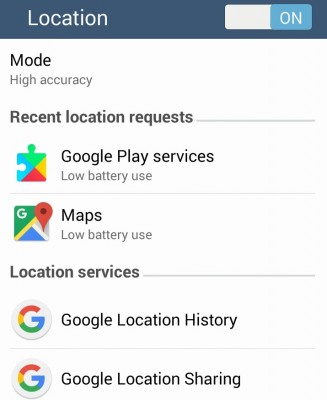This screenshot displays a section of a smartphone screen dedicated to location settings. Although the smartphone's top header is not visible, the top part of the screen is highlighted by a navy blue background. On the left side of this background, the word "Location" is written in white, while on the right side, a rectangular switch shows a dual-colored background—half white and half light blue—with the word "ON" in capital letters on the light blue side.

Immediately below, the screen's main background shifts to white. At the upper left corner, the word "MODE" is written in black font. Beneath this heading, the option "High Accuracy" is displayed in gray font. Further down, a section titled "Recent Location Requests" is shown in dark gray font, listing recent apps that have requested location data.

The first app listed is "Google Play Services," identifiable by its older logo, which resembles a jigsaw puzzle piece colored in blue, green, yellow, and red. Below this, "Maps" is listed, marked by its erstwhile logo featuring a red location marker and a square sectioned into green, blue, and white quarters.

Further down, a section titled "Location Services" appears. Under this heading, two entries are listed. The first is "Google Location History" accompanied by the Google 'G' logo in red, yellow, green, and blue. The second is "Google Location Sharing," also denoted by the Google 'G' logo to the left.